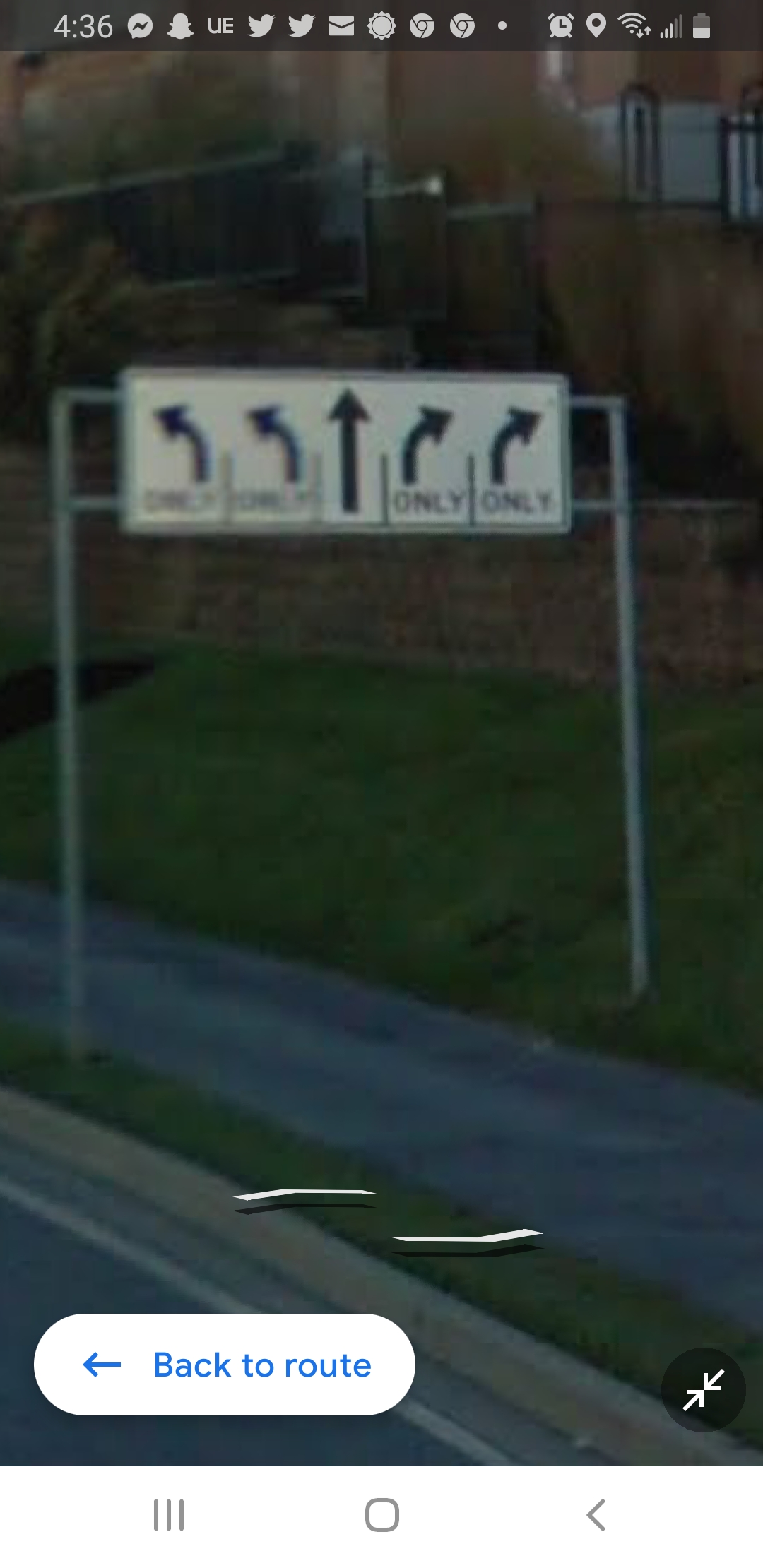This image is a detailed screenshot of a Google Maps interface. Prominently featured in the center of the screen is a road sign pole that spans from one side of the road to the other. Attached to the pole is a large sign displaying various navigational instructions. In the middle of the sign, there is a straightforward arrow indicating to proceed straight. On either side of this central arrow, there are two arrows pointing left and right respectively, which signify turning options. Additionally, at the top left corner of the sign, there is a small blue arrow labeled "Back to Route."

The screenshot also captures the user's notification bar at the top of the screen. The notifications reveal that several apps are currently open: Messenger, Twitter, two instances of Google Chrome, and an alarm clock app. Indicators show the user’s location services are active, the Wi-Fi signal is strong, and the battery level is at half capacity. The current time displayed is 4:36.